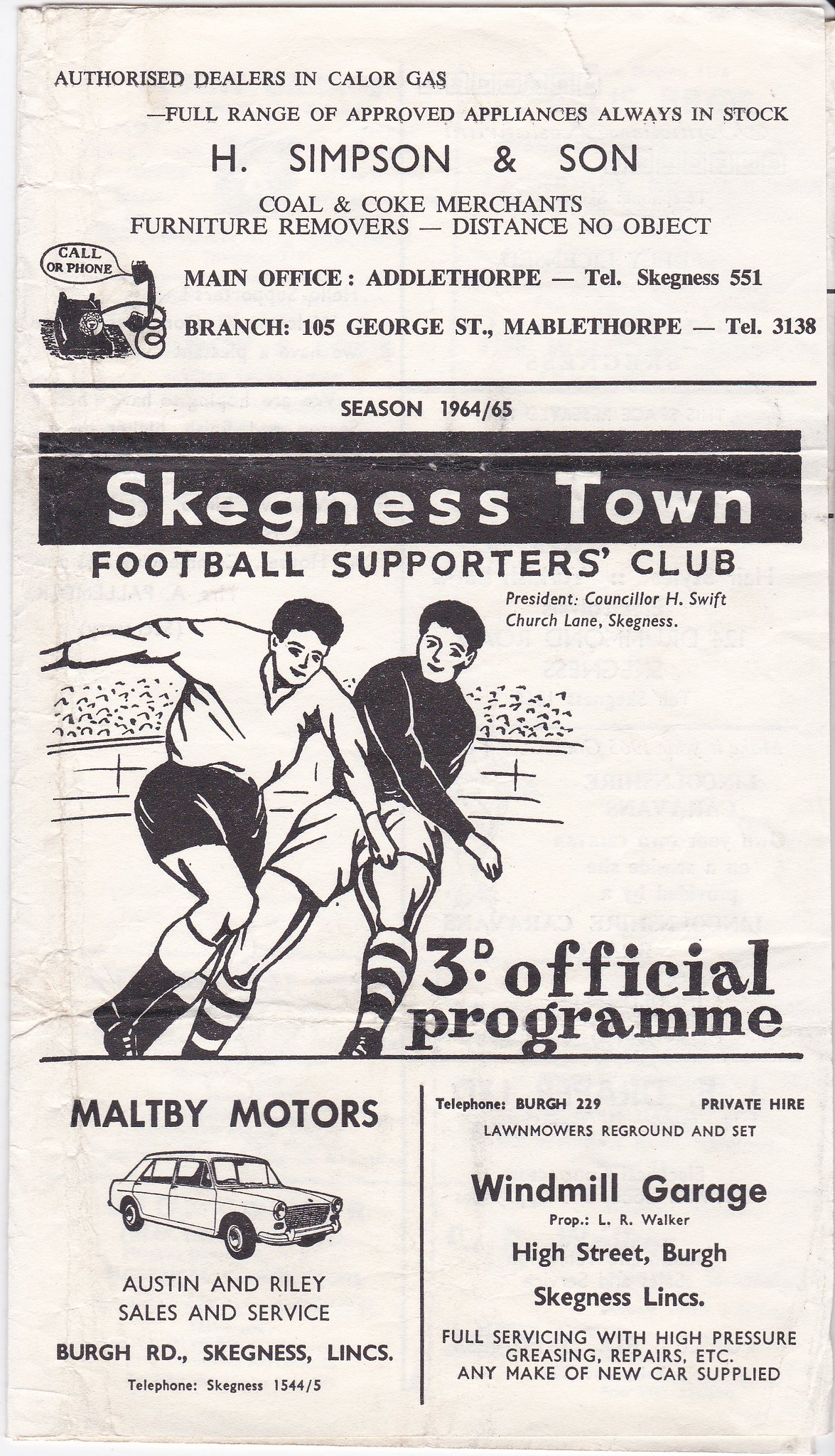This black-and-white photograph captures the cover of an official football program from the 1964-65 season for the Skegness Town Football Supporters Club. The page, from an old magazine or newspaper, is divided into three main sections. 

The top section features an advertisement for H. Simpson and Son, identified as authorized dealers in various appliances, including Collar Gas, and suppliers of coal and coke, as well as providing furniture removal services. The midsection sports a hand-drawn illustration of two soccer players vying for the ball amidst a doodled background of a cheering crowd. Prominently displayed around the illustration is the title "Skegness Town Football Supporters Club" along with text stating "Official Program" and "Season 1964 to 65." A note mentions the president as Counselor H. Swift. 

The bottom section contains two advertisements. On the left, an ad for Maltby Motors showcases an image of a sedan, promoting Austin and Riley Sales and Services. The right side features an ad for Windmill Garage, highlighting services such as lawnmower regrinding, high-pressure greasing, and repairs, and noting that they can supply any make of new car. This elaborate cover provides a nostalgic glimpse into the local football culture and businesses of 1960s England.